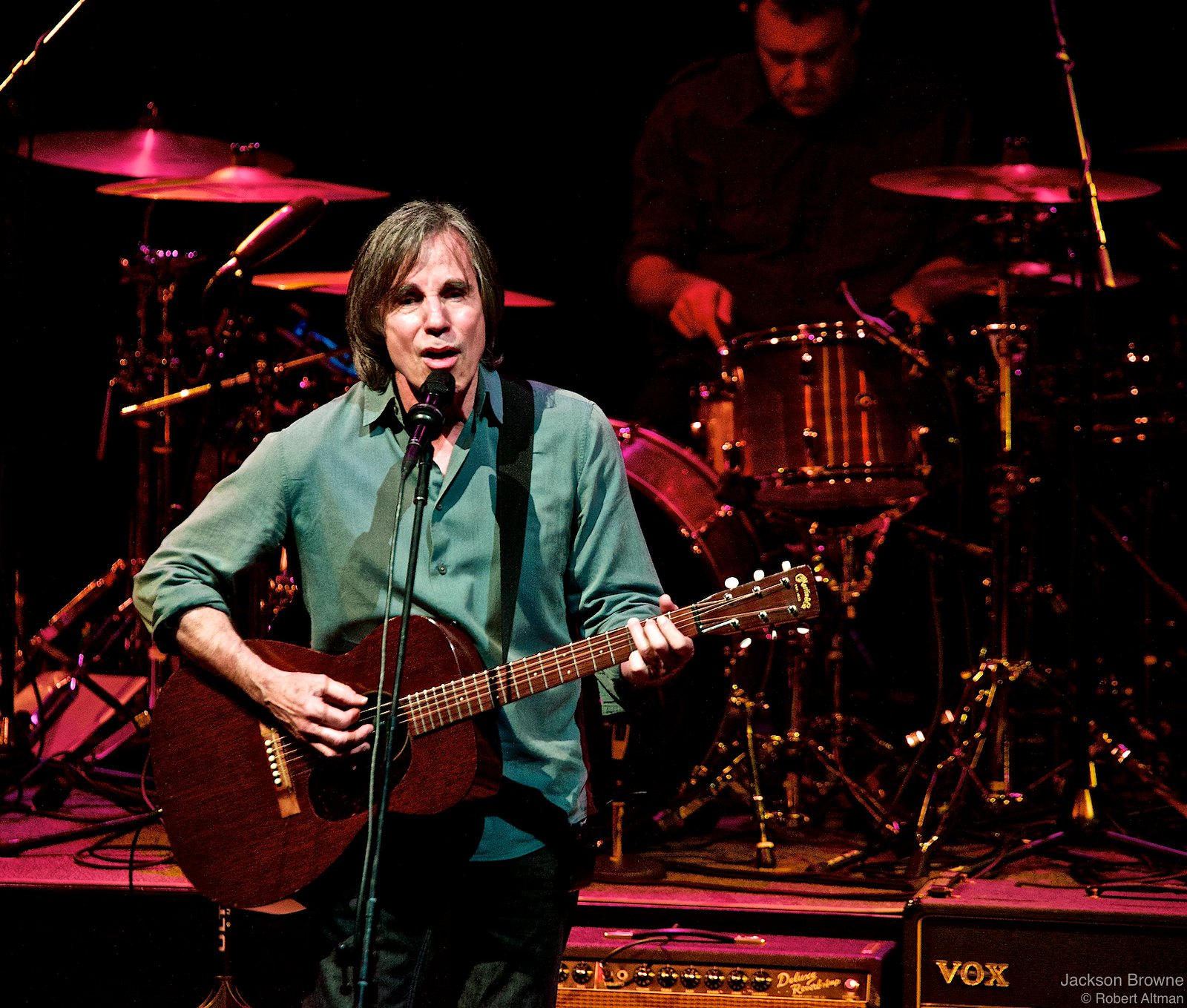The image features the renowned musician Jackson Browne performing on stage. Positioned slightly off-center to the right, Jackson is captured strumming a dark mahogany acoustic guitar. He is dressed in a light green button-down shirt and dark jeans. His long hair, exhibiting shades of brown and gray, falls over his ears and down to his neck. He is gazing intently at the background, possibly connecting with his performance.

Behind him, a drummer is actively engaged with the drum set, which comprises various components including snare and bass drums as well as cymbals. The drum set predominantly displays hues of brown, silver, and black, and the drummer's focused demeanor is evident as he looks down at his instrument. Additionally, large amplifiers, one of which is branded "Vox," can be seen between Jackson and the drummer.

The stage is enveloped in a dark, moody ambiance with light and shadow playing across the instruments and Jackson's figure. Hints of red lighting cast a warm glow onto the stage setup, enhancing the overall atmosphere. A microphone in front of Jackson signifies his role as the lead singer, serenading the audience. The bottom corner bears the note: "Jackson Browne copyright Robert Almond," confirming the artist's identity.